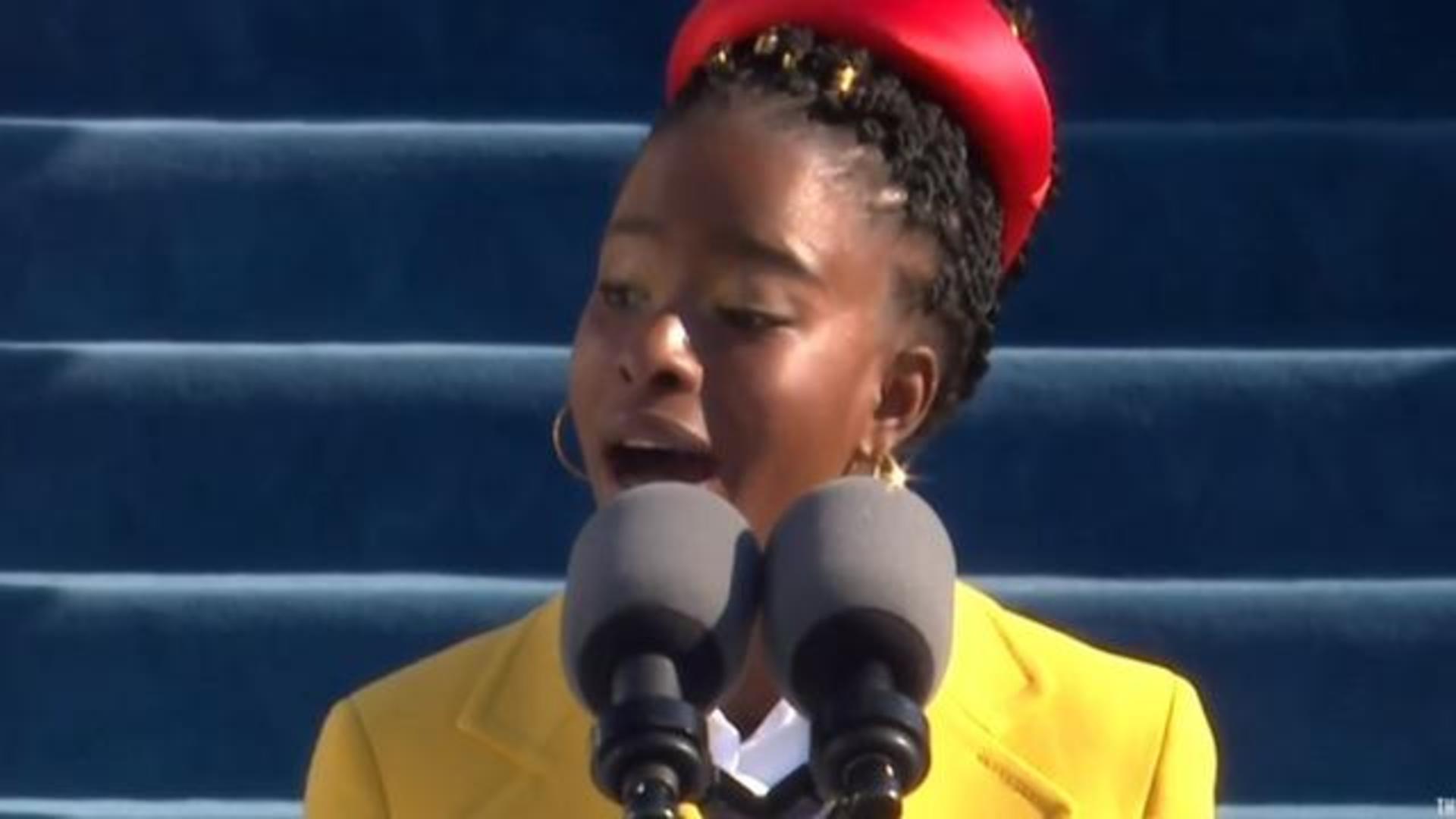This image features a young African American woman speaking at the recent presidential inauguration. She stands behind two large gray microphones equipped with wind guards. Her attire is striking, consisting of a bright yellow coat over a white blouse, complemented by a red satin or leather pillbox hat. She accessorizes with gold hoop earrings and an elaborate braided hairstyle adorned with gold jewels or beads. The backdrop includes a set of deep blue carpeted stairs that catch the sunlight, adding a gradient effect. The woman, with her body facing forward and head turned slightly to the right, gazes intently to the side, her expression a mix of nostalgia and passion. The tight framing of the photo focuses on her from the shoulders up, emphasizing her poised presence and the significance of the occasion.